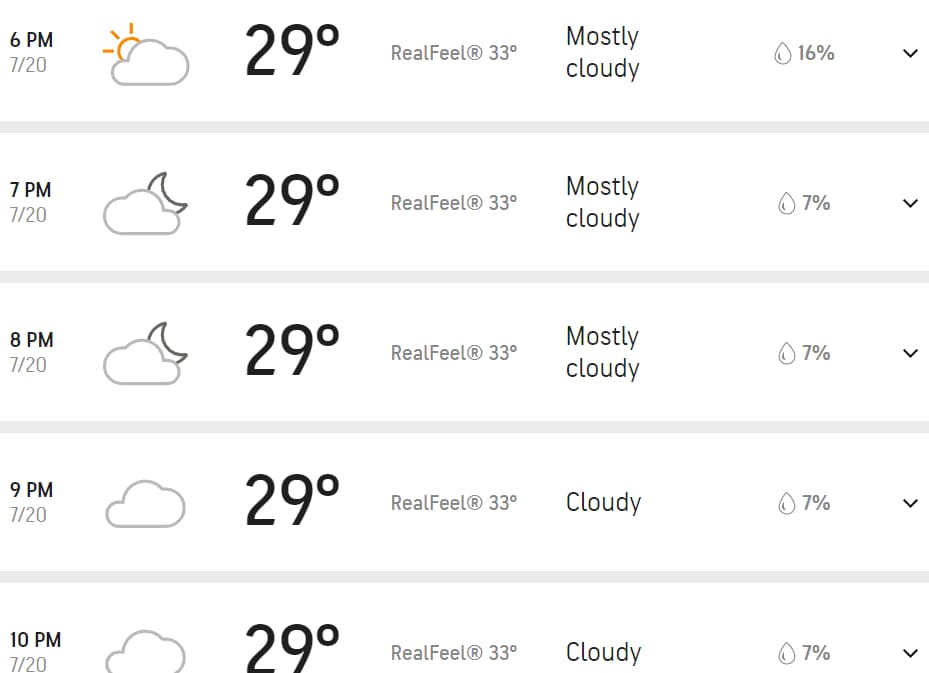This image is a screenshot from a mobile weather application displaying the hourly weather forecast for the evening of July 20th. The forecast spans from 6 p.m. to 10 p.m. with detailed weather conditions listed for each hour. At 6 p.m., the weather is partly cloudy with an estimated temperature of 29°C, a real feel of 33°C, and a 16% chance of precipitation. By 7 p.m., the sun has set, and the weather is mostly cloudy, maintaining the same temperature and real feel, but with a reduced 7% chance of precipitation. This trend continues through 8 p.m., 9 p.m., and 10 p.m., where the temperature remains consistent at 29°C with a real feel of 33°C. The cloud coverage increases to fully cloudy from 9 p.m. onwards, with a persistent 7% chance of precipitation. The app's interface features a plain white background, keeping the focus on the weather details.